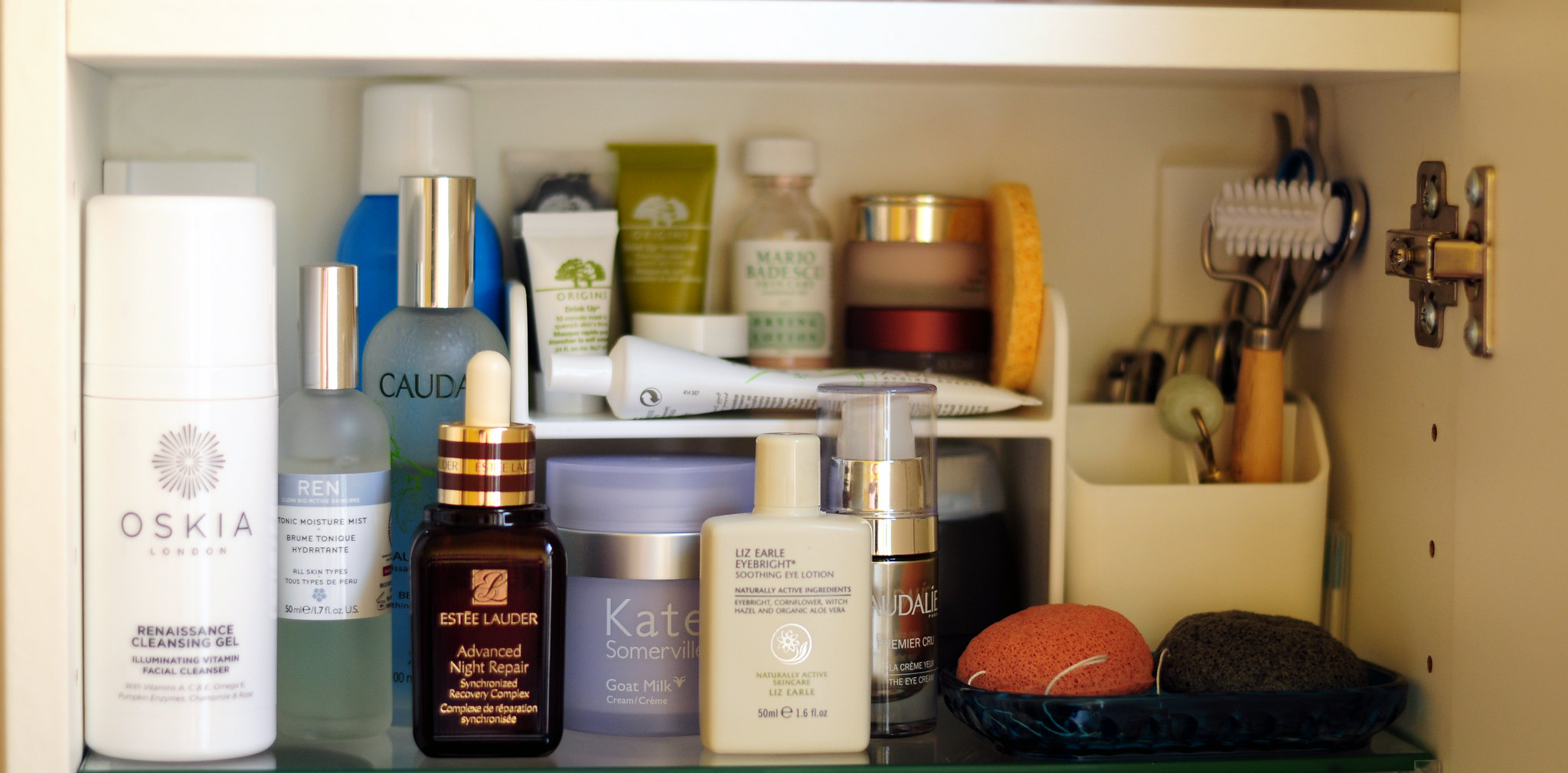The image captures the bottom shelf of a white medicine cabinet, with a zoomed-in focus on the details. A brass hinge is visible on the right side of the cabinet, accompanied by three small holes beneath it. The shelf is populated primarily on the left side with an array of twelve to fifteen personal care items, including perfumes, makeup, and cleansing gels, which extend about three-quarters of the way towards the right.

Prominently featured on the far left is an Oskia cleansing gel, housed in a white bottle displaying a floral label and the brand name "Oskia" in purple font. Adjacent to it is a dark brown bottle of Estee Lauder Advanced Night Repair. A smaller purple container by a brand named Kate is situated nearby, along with a neighboring bottle of brownish cream. An Estee Lauder perfume bottle is placed next to these. More towards the back of the shelf are several smaller bottles, adding to the diverse assortment.

On the right side of the shelf, a bin holds a few grooming tools. Among these tools is a particularly noticeable one with an orange handle and a white brush head with small spikes. This detailed composition reveals a well-stocked and organized section of the medicine cabinet.